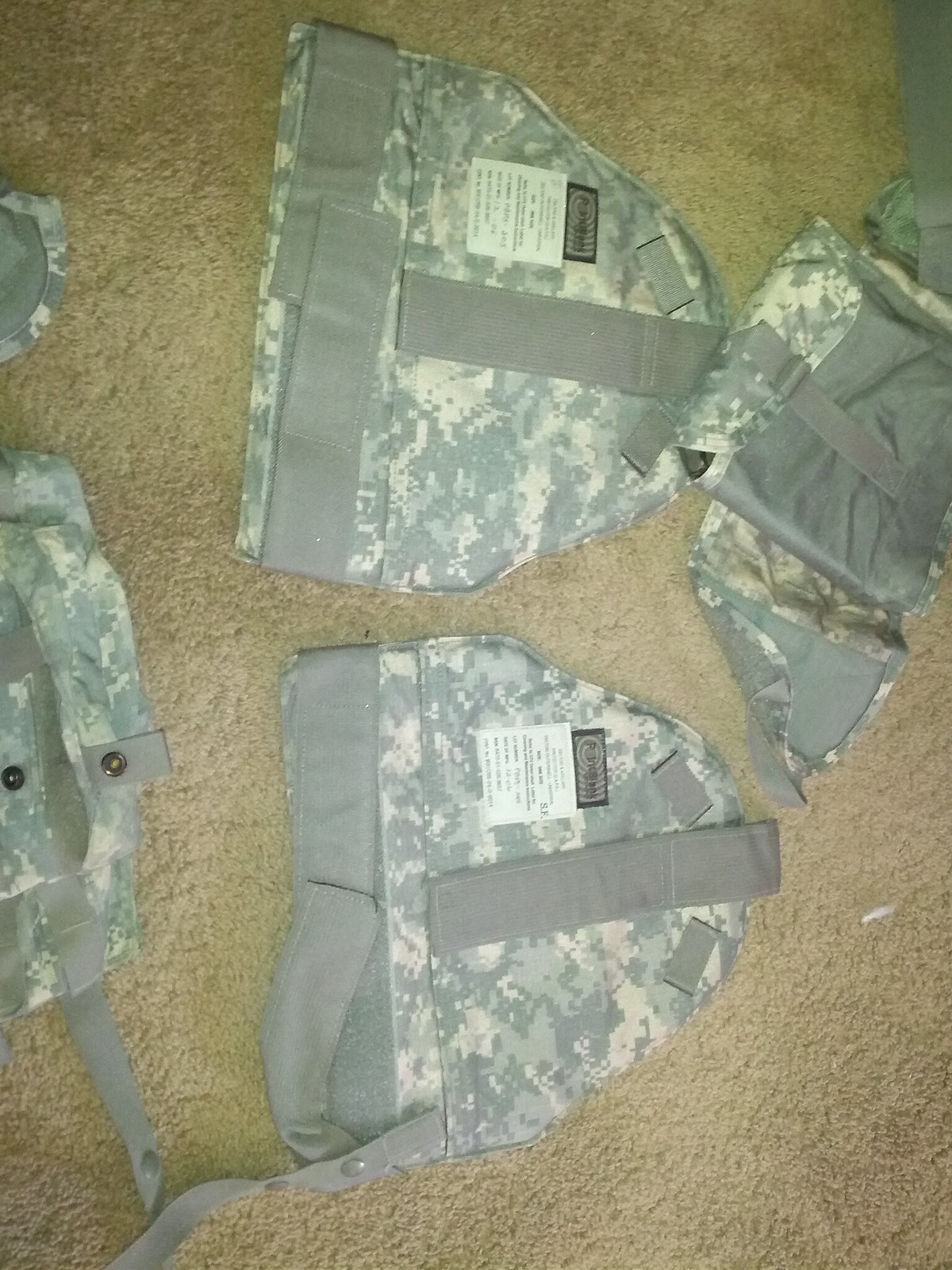This is a detailed top-down photograph in portrait mode, showcasing various items of military or hunting gear laid out on a light beige carpet. Central to the image are two camouflage caps resembling beanie-style hats, adorned with green, gray, and white patterns and featuring Velcro and light green or gray trim around their headbands. Surrounding these are four additional items in similar camouflage colors. To the top right, there appears to be a belt or strap outfitted with pockets and snaps. On the left side, two more objects are partially visible, one small and indistinct, the other resembling a bag with Velcro and poppers. The image captures the textured, light brown carpet as the backdrop for displaying this collection of military-themed gear.